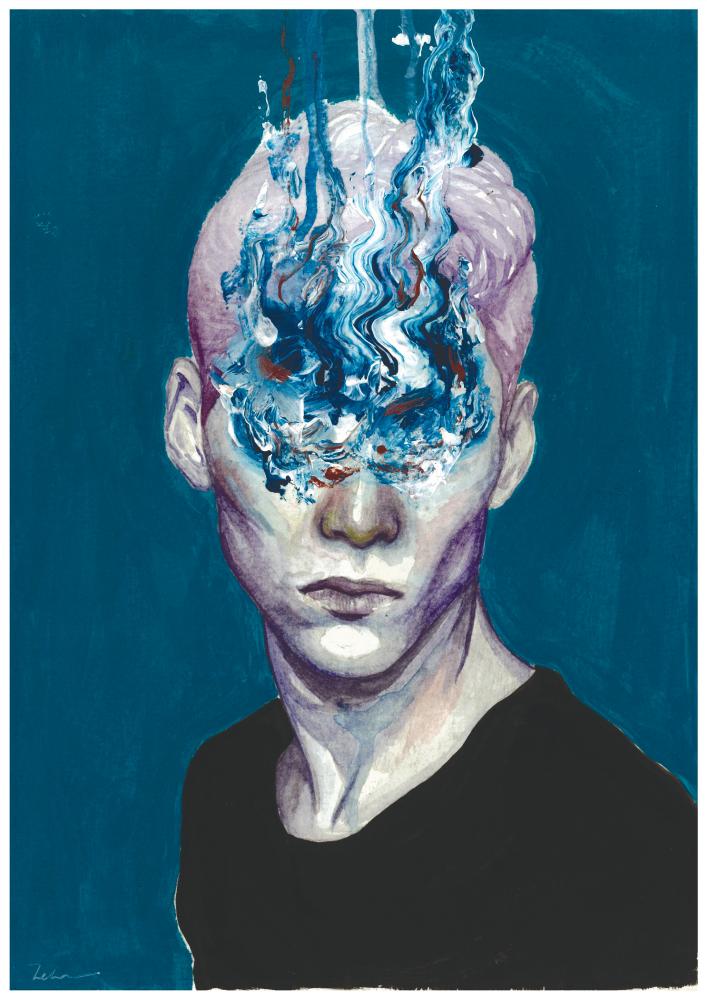This watercolor painting features a thin man standing against a dark blue background that fades to a lighter blue towards the bottom. The man is depicted with fair skin, sallow cheeks, and a frowning expression. He is wearing a black T-shirt with a scoop collar and is turned slightly to the right, his head facing directly toward the artist. His posture shows one shoulder arched with the other dropped back, creating a dynamic, almost tense pose. His hair is a striking pinkish-purple color, partially obscured by an abstract, fiery distortion around his eyes. This eye area is depicted with swirling, smoke-like lines in shades of blue, white, and maroon that rise past his hair and blend into the background. The eyes are entirely obscured by this wavy, mask-like formation, creating an effect as though the facial area from the middle of the nose upwards is melting or on fire. The distortion captures attention, creating a surreal, almost haunting focal point in the artwork.